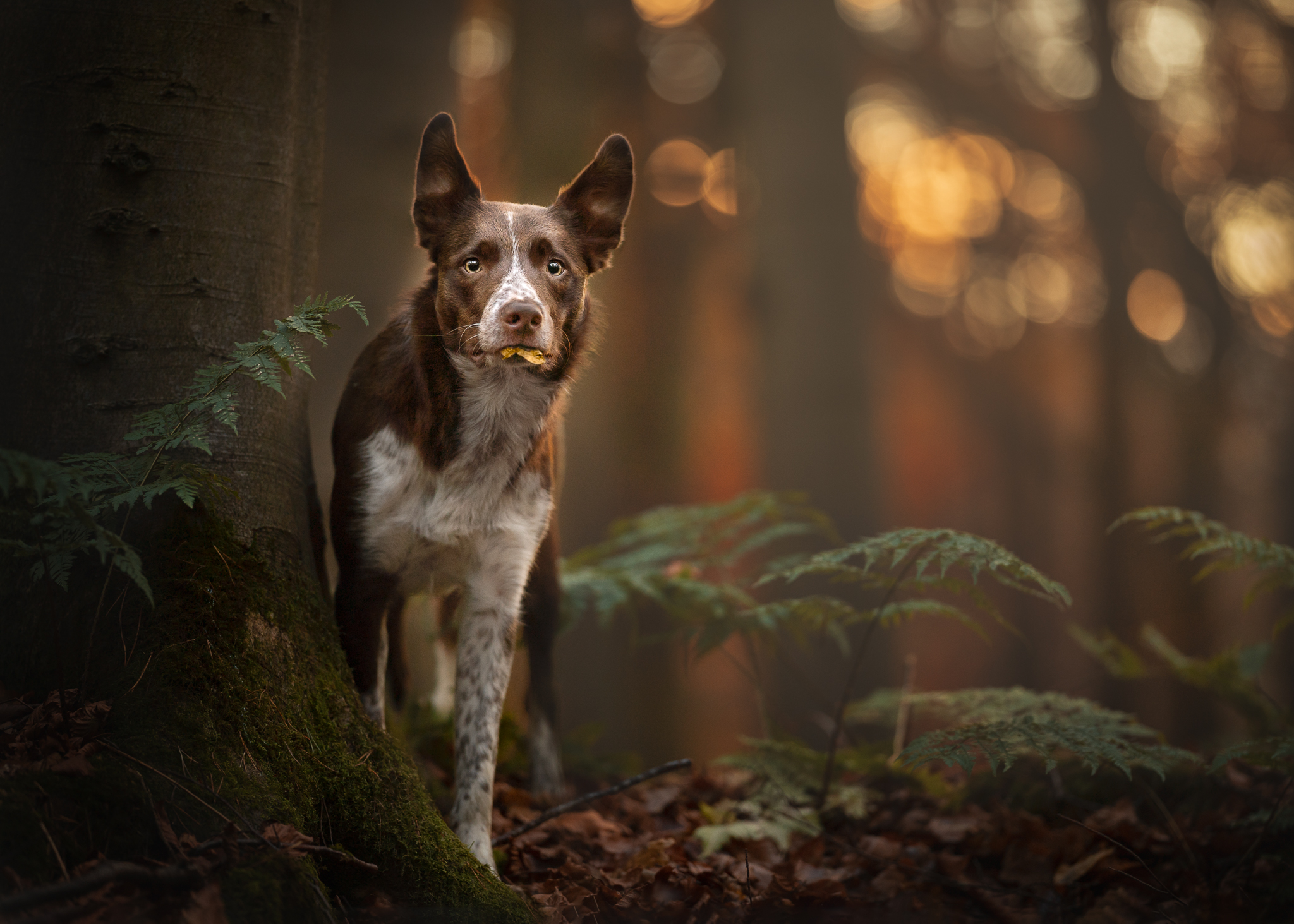This is an extremely high-resolution photograph of a beautiful dog, possibly a spaniel or a hunting dog, standing in the middle of a vibrant, forested area. The dog has striking brown fur with a white chest and white paws speckled with brown, and its face is predominantly brown with white across the muzzle adorned with brown freckles. Its expressive, wide, light brown eyes look scared and are directed straight at the camera. Its tall, erect ears frame its face, and the dog holds a yellow leaf in its mouth.

The setting appears to be a brown forest during dusk, with amber sunlight filtering through the trees, creating a dreamy, soft brown light in the background. The forest floor is covered with various brown and orange leaves, bright green ferns, and a dark brown tree trunk with green moss at its base. The backdrop features yellowish and white light dots, adding to the vibrant atmosphere of this serene outdoor scene.